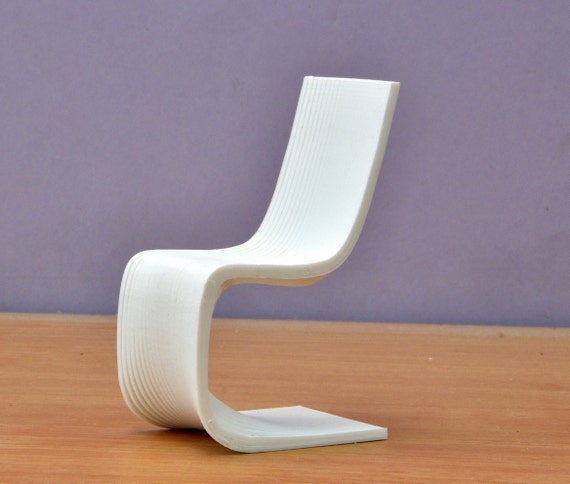This image showcases a very modern and futuristic chair, positioned on a light brown wooden floor. The background features walls painted in a light purple, almost lilac, color that dominates the scene. The chair is constructed from a solid piece of white, molded plastic and boasts an intriguing, ribbed texture throughout its surface. 

From a side view, the chair curves in a continuous, fluid motion: it begins at the lower back, swooping downward like a waterfall, then transitions smoothly forward to form the seat before curving down again and finally bending back underneath, resembling the shape of a 'C' or 'D'. The back of the chair is subtly tilted backward, which suggests a slightly reclined seating position. The overall design is both clean and artistic, with the chair facing left and a bit towards the front, adding to its dynamic and modern aesthetic.